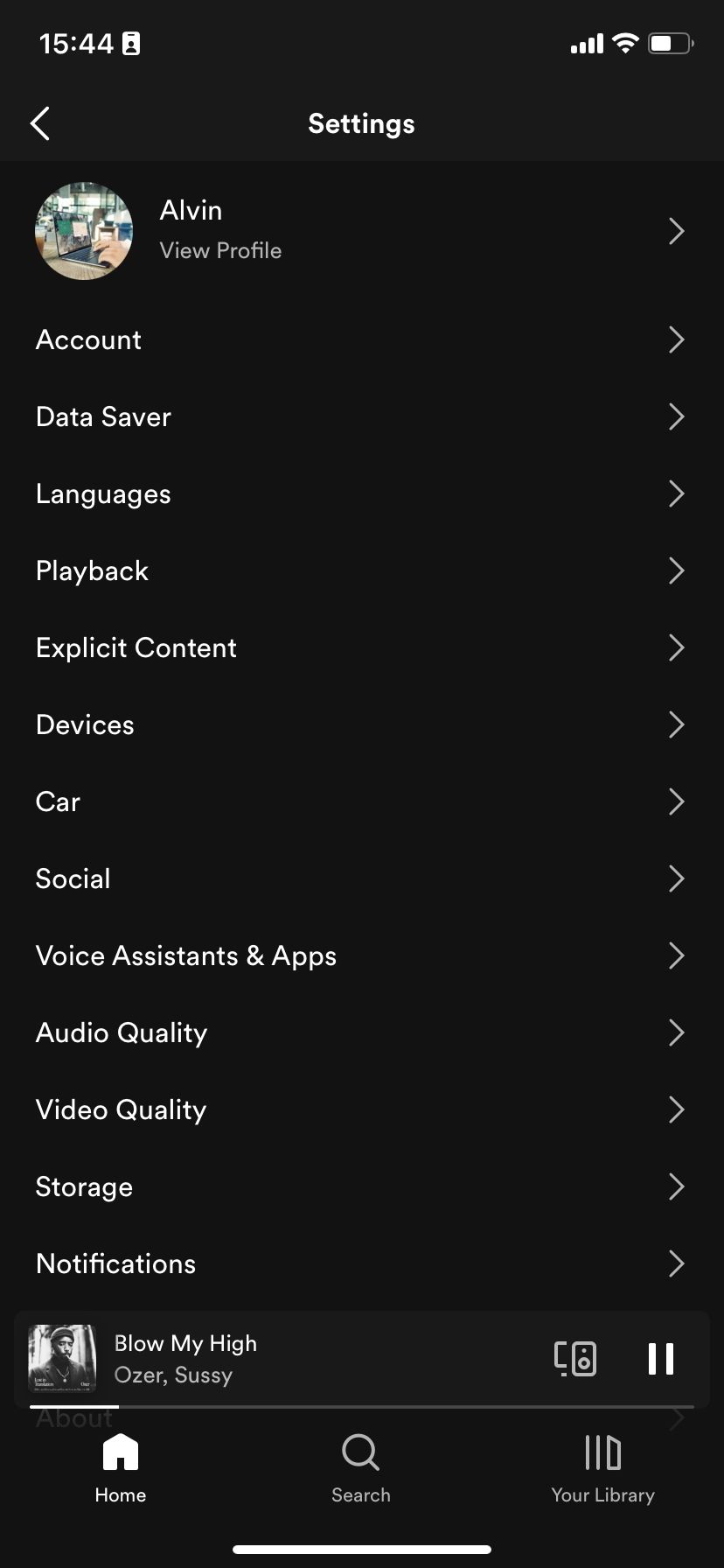Title: Detailed Overview of Spotify Settings on Mobile

Caption:
This image captures a detailed screenshot of the Spotify settings section on a mobile phone, prominently featuring a sleek black background consistent with Spotify's dark theme. The status bar of the mobile phone, also black, seamlessly blends with the settings interface.

Dominating the top section of the settings is the profile header featuring Alvin. His avatar, depicting him typing on a laptop, is accompanied by his name. Below Alvin’s profile, there is an "Account" line, followed by an extensive list of settings options including "Data Saver," "Languages," "Playback," "Explicit Content," "Devices," "Car," "Social," "Voice Assistance and Apps," "Audio Quality," "Video Quality," "Storage," and "Notifications."

Notably, this settings section is specific to the Spotify app rather than the mobile phone’s general settings. At the bottom of the screenshot, the currently playing song "Blow My High" by Ozur Hussey is displayed, showcasing Spotify's player interface. The footer includes three essential navigation buttons: a 'Home' button, a 'Search' button, and a 'Library' icon, all vital for navigating through the app.